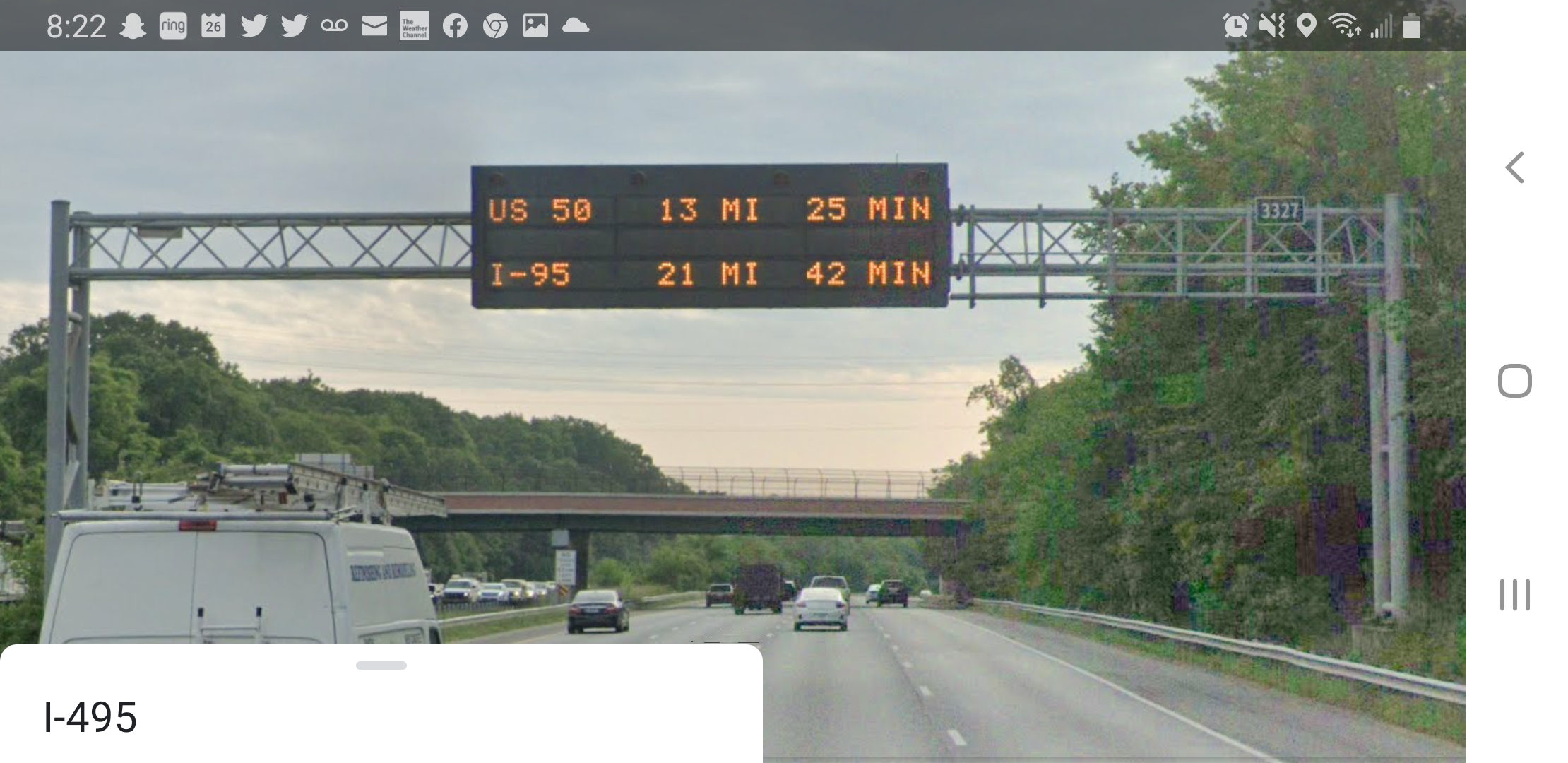This screenshot, likely captured from a dash cam or tablet, features a highway scene on I-495. The device's status bar is visible at the top, displaying common icons such as a battery indicator on the right, and Wi-Fi and signal strength indicators on the left. The current time, shown as 8:22, is also visible alongside app icons for Twitter, Snapchat, email, and Facebook. The image centers on a highway sign and a bridge in the distance. The road is framed by lush, green trees on both sides and populated with several vehicles, including a notable van with a ladder mounted on its side, positioned to the left of the car from which the image is taken.